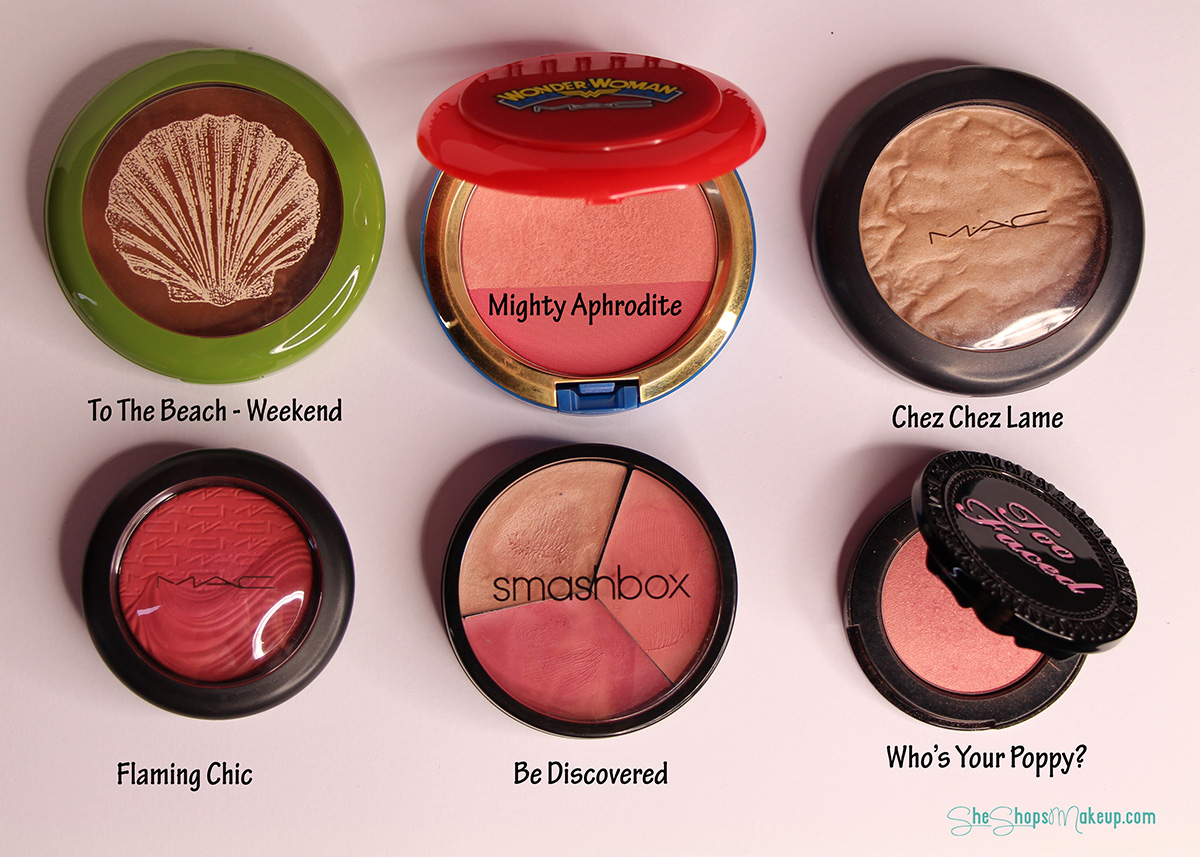The image displays six round makeup compacts neatly arranged on a light pink table. The first top-left compact features a green case with a tan seashell design, labeled "To the Beach - Weekend." Next to it, on the right, is an open compact with a red lid that has yellow writing, reading "Wonder Woman" along with the winged Wonder Woman logo, and inside it says "Mighty Aphrodite." The third compact on the top row is black and closed, marked with the brand MAC and the name "Shea Shea Lame." On the bottom row, directly beneath the seashell compact, is another MAC compact, this one pink and labeled "Flaming Chic." Next to it, in the middle, is a Smashbox compact divided into three pie-chart-like sections in various pink shades, labeled "Be Discovered." The last compact to the right is black and open, with pink makeup inside; it is a Two Faced product with the inscription "Who's Your Poppy" on the inner lid.